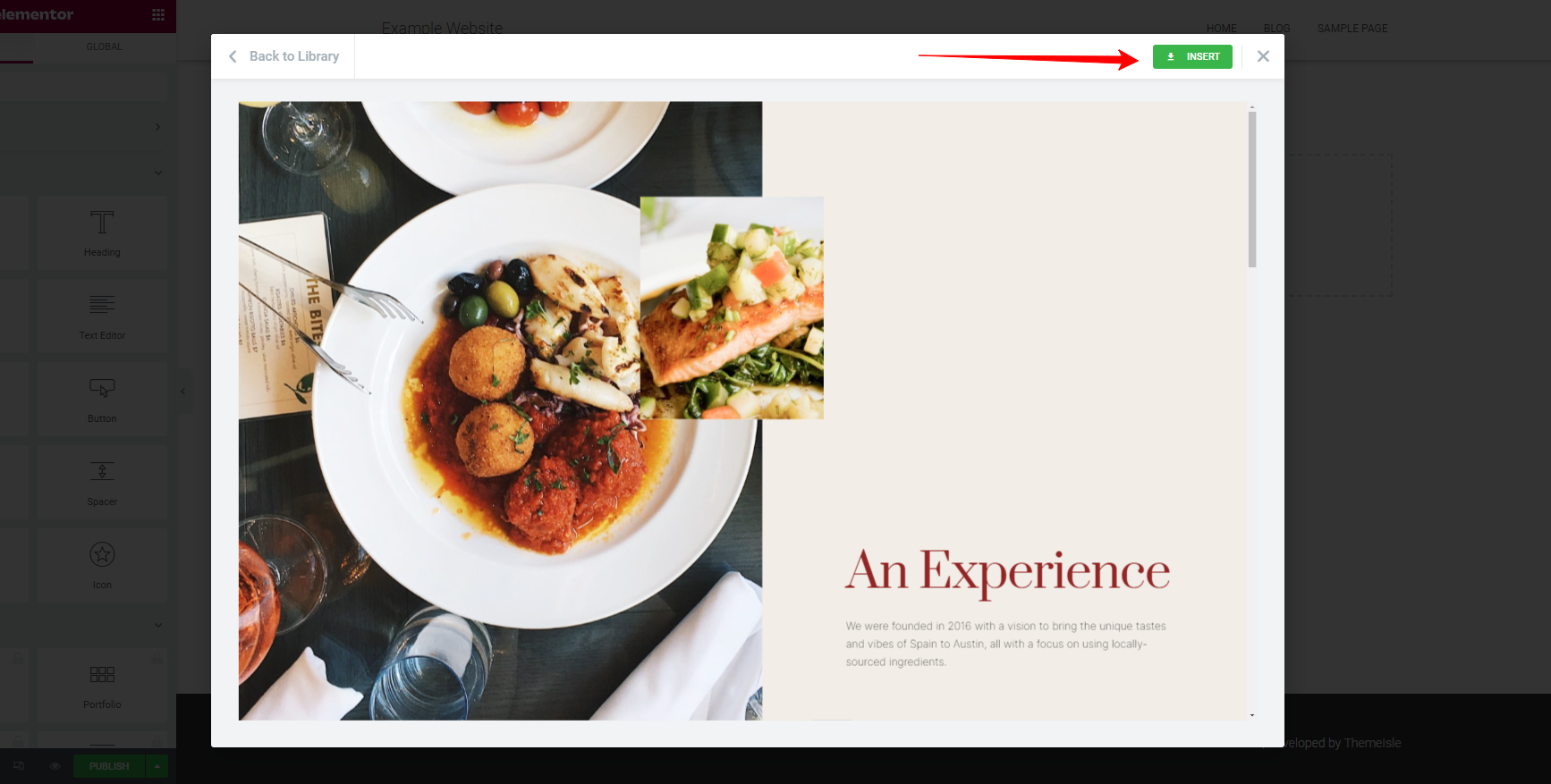In this image, we observe a pop-up window displayed on a computer screen. The upper left corner of the pop-up features a button labeled "Back to Library," while the upper right corner contains an 'X' button for closing the window. A prominent green button, possibly for downloading, is located on the right side of the pop-up, highlighted by a red arrow that has been added to the image to draw attention to this button.

The main body of the pop-up is occupied by a block of text positioned near the bottom right, which reads, "An experience we were founded in 2016 with the vision to bring the unique tastes and vibes of Spain to Austin, all with a focus on using locally sourced ingredients."

On the left side of the pop-up, there are two images of food. The lower image depicts a plate containing a sauce-covered dish with meatballs, while the upper image appears to showcase a dish of salmon or another type of fish, accompanied by vegetables on top. In the background of the pop-up, the interface of the website used to build this site is faintly visible.